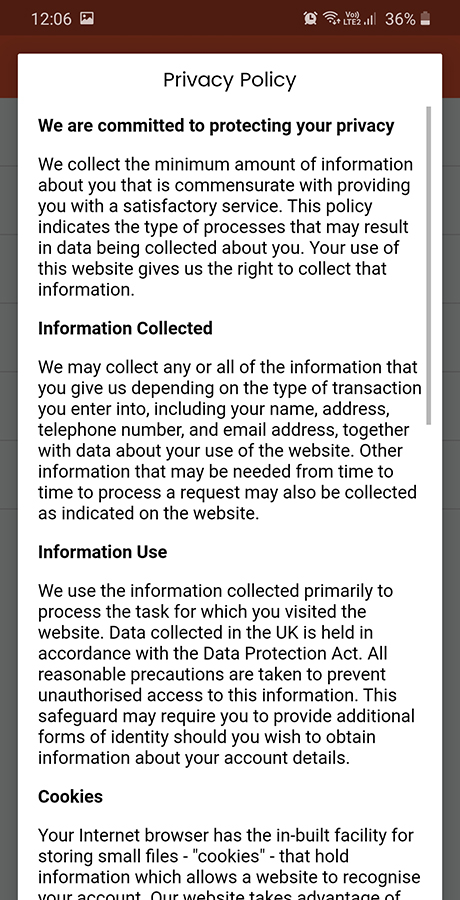A detailed image description for a cell phone screen displaying a privacy policy notification:

The image shows a smartphone screen with the current time displayed as 12:06 in the upper left corner. The status bar next to the time shows several icons: an alarm clock, signal bars for cellular data, signal bars for cellular reception, and a battery icon indicating 36% charge remaining. 

The top section of the screen is filled with a red background that transitions to gray at the bottom. Overlaying this is a prominent white rectangular notification that is vertically oriented and occupies a significant portion of the screen. 

The notification is a privacy policy statement that reads:

_"Privacy Policy: We are committed to protecting your privacy. We collect a minimum amount of information about you that is commensurate with providing you a satisfactory service. This policy indicates the type of processes that may result in data being collected about you. Your use of this website gives us the right to collect that information."_

_"Information Collected: We may collect any or all of the information that you give us depending on the type of transaction you enter into, including your name, address, telephone number, email address, together with data about your usage of the website. Other information that may be needed from time to time to process a request may also be collected as indicated on the website."_

_"Information Use: We use the information collected primarily to process the tasks which you have visited the website for. Data collected in the UK is held in accordance with the Data Protection Act. All reasonable precautions are taken to prevent unauthorized access to this information. The safeguard may require you to provide additional forms of identity should you wish to obtain information about your account details."_

_"Cookies: Your internet browser has a built-in facility for storing small files, i.e., 'cookies,' that hold information which allows the website to recognize your account."_

This visual description captures all the details of the cell phone's user interface and the privacy policy that is currently being displayed.